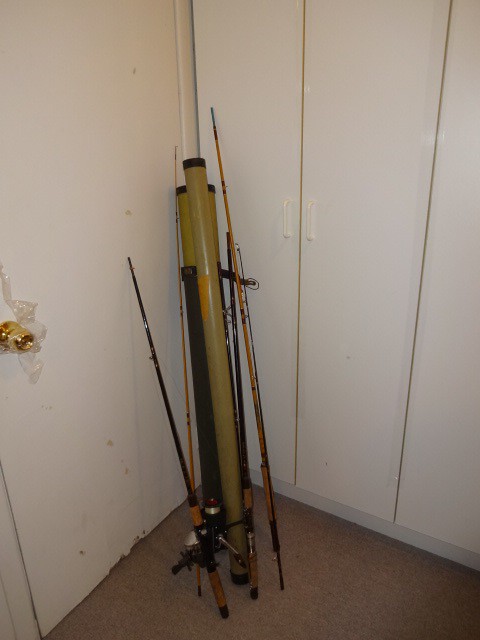The photograph depicts the corner of a white-walled room, where a white door with a golden handle occupies the left side. At the base of this door, there is a noticeable section of broken wood. On the right side, there is a built-in white cabinet with small, rounded handles in the center of the doors. The floor is carpeted in brown. Leaning against the corner where the door meets the cabinet are several fishing poles and their containers. The fishing poles, which vary in height and color, include shades of beige and black, with some marked by an orange-yellow hue and brown accents. There are also three cylindrical olive-green containers, seemingly designed to hold fishing gear, placed among the fishing poles. The collection includes approximately six or seven items, such as poles and containers, with one fishing pole equipped with a reel.